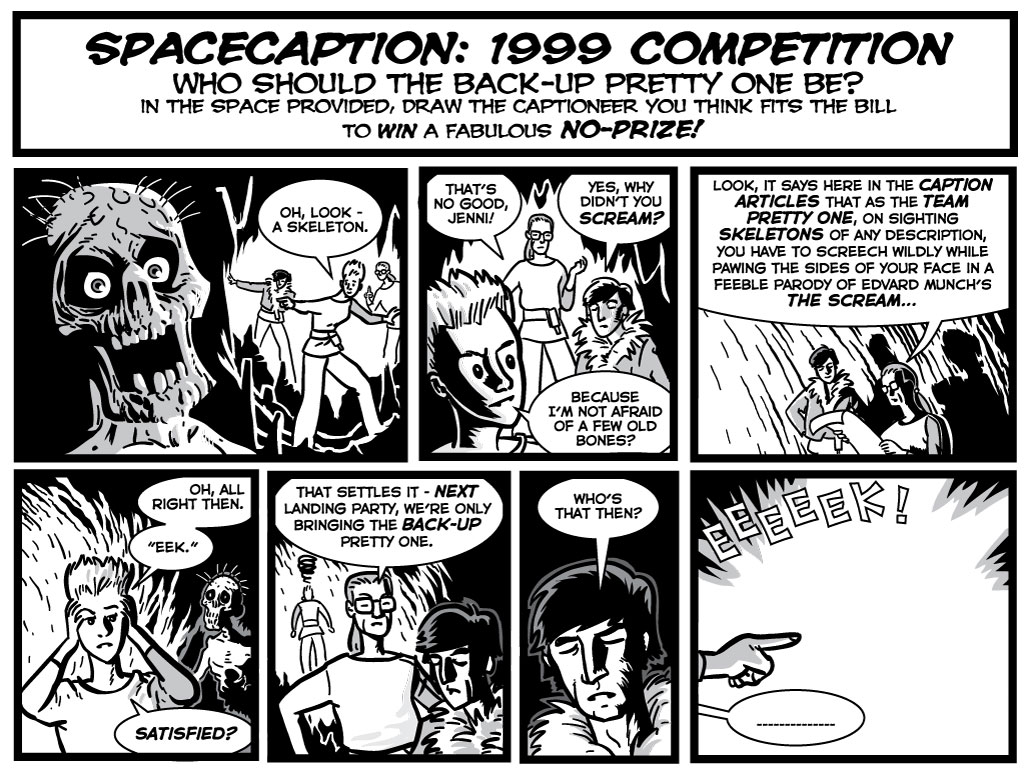The image is a horizontally aligned rectangular comic strip presented in black and white, titled "SPACE CAPTION: 1999 COMPETITION" in bold, all-caps letters at the top. Just below this, a smaller-font question asks, "Who should the backup pretty one be?" This is followed by an instruction stating, "In the space provided, draw the captioneer you think fits the bill to win a fabulous no prize!"

The comic strip is divided into two rows of panels—three on the top and four on the bottom, all varying in size and shape. The first upper-left panel features a screaming skeleton or skull. To the right of this, another panel shows a group of three men noticing the skeleton, with one exclaiming, "Oh, look, a skeleton." Moving further right, another panel captures the same group discussing the situation, with dialogue such as, "That's no good, Jen. Yes, why didn't you scream?" Near the end of the top row, the men continue their conversation, and the last panel shows one holding a paper.

In the bottom row, the narrative continues with the men conversing, reacting, and showing various emotions. At one point, a character confidently declares, "Because I'm not afraid of a few old bones." Panels towards the center show the group further deliberating, and the final bottom-right panel climaxes with a loud "Eek!" directed at yet another surprising revelation.

Overall, the comic exudes a mixture of suspense and humor as the characters react to the eerie but somewhat humorous scenario involving the skeleton.